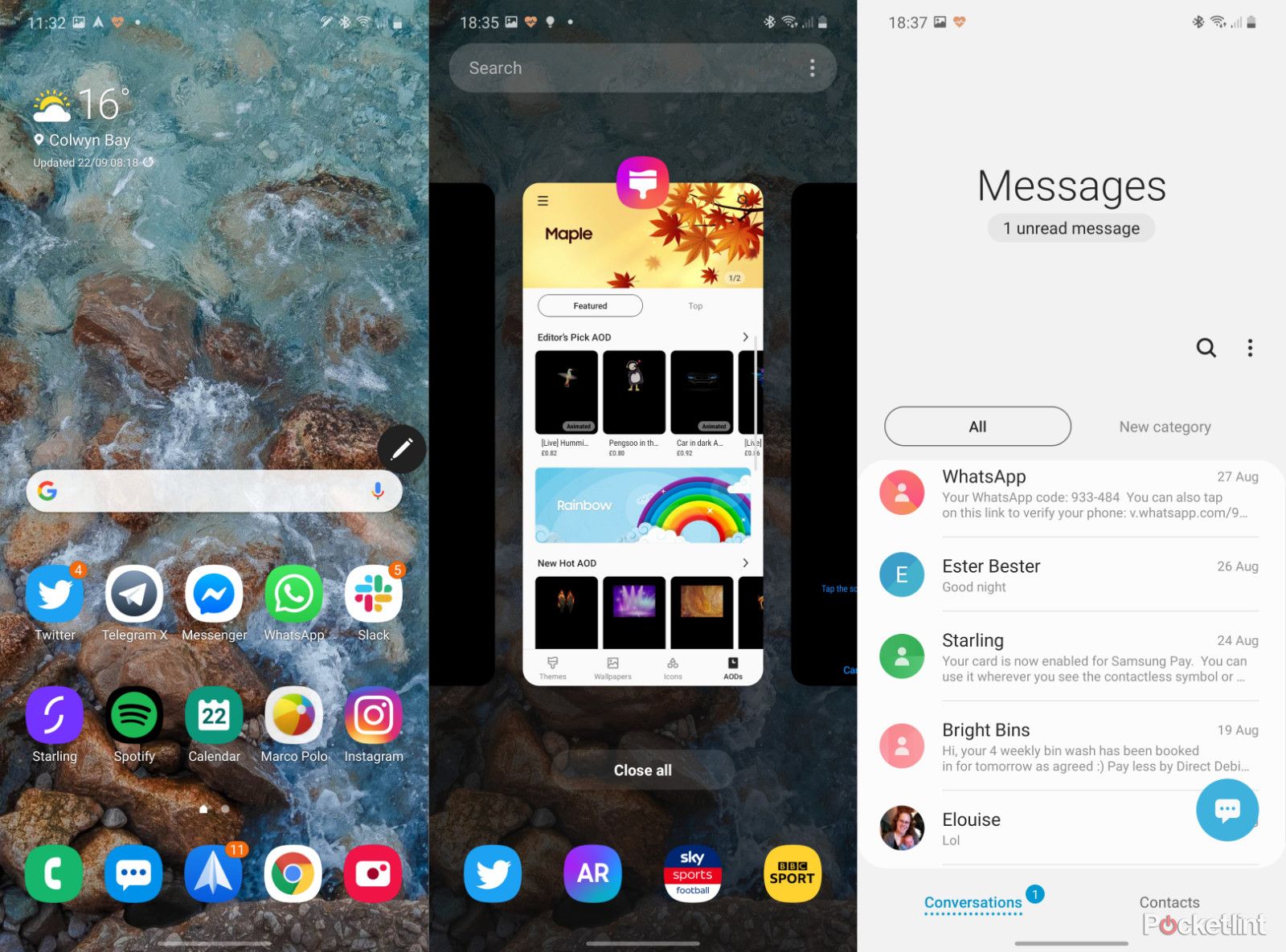The image consists of three seamlessly connected cellphone screenshots presented side by side, without any borders or gaps between them.

- **Left Screenshot**: This screenshot showcases a cellphone wallpaper depicting an oceanic scene with rocks. The time displayed on the screen is 11:32 AM, and the weather information indicates it is partly sunny with a temperature of 16 degrees in Colwyn Bay. Prominently featured is a Google search bar, below which are a selection of app icons including Twitter, Telegram X, Messenger, WhatsApp, Stack, Slack, Google, a telephone icon, and Instagram.

- **Center Screenshot**: The central screenshot has a dark, somewhat indistinct background with the time shown as 6:35 PM. A gray search bar is positioned at the top. The middle portion displays an image of a phone screen with the word "Maple" inside a yellow rectangle at the top. Further down, a motif of leaves is visible, alongside some musical elements. It mentions "Editor's pick AOD" and includes other text like "live something" (difficult to read). There's also a white background area featuring a picture of a rainbow labeled "rainbow." Near the bottom are black boxes labeled "New Hot AOD."

- **Right Screenshot**: The rightmost screenshot has a predominantly gray theme and shows a messaging interface under the title "Messages." Within this interface are several conversation entries, each represented with a circular icon. The visible contacts include WhatsApp symbols, Esther Better, Starling, Bright Bins, and Eloise—accompanied by a thumbnail image of Eloise.

This detailed arrangement provides a comprehensive visual summary of the three interconnected cellphone screenshots.